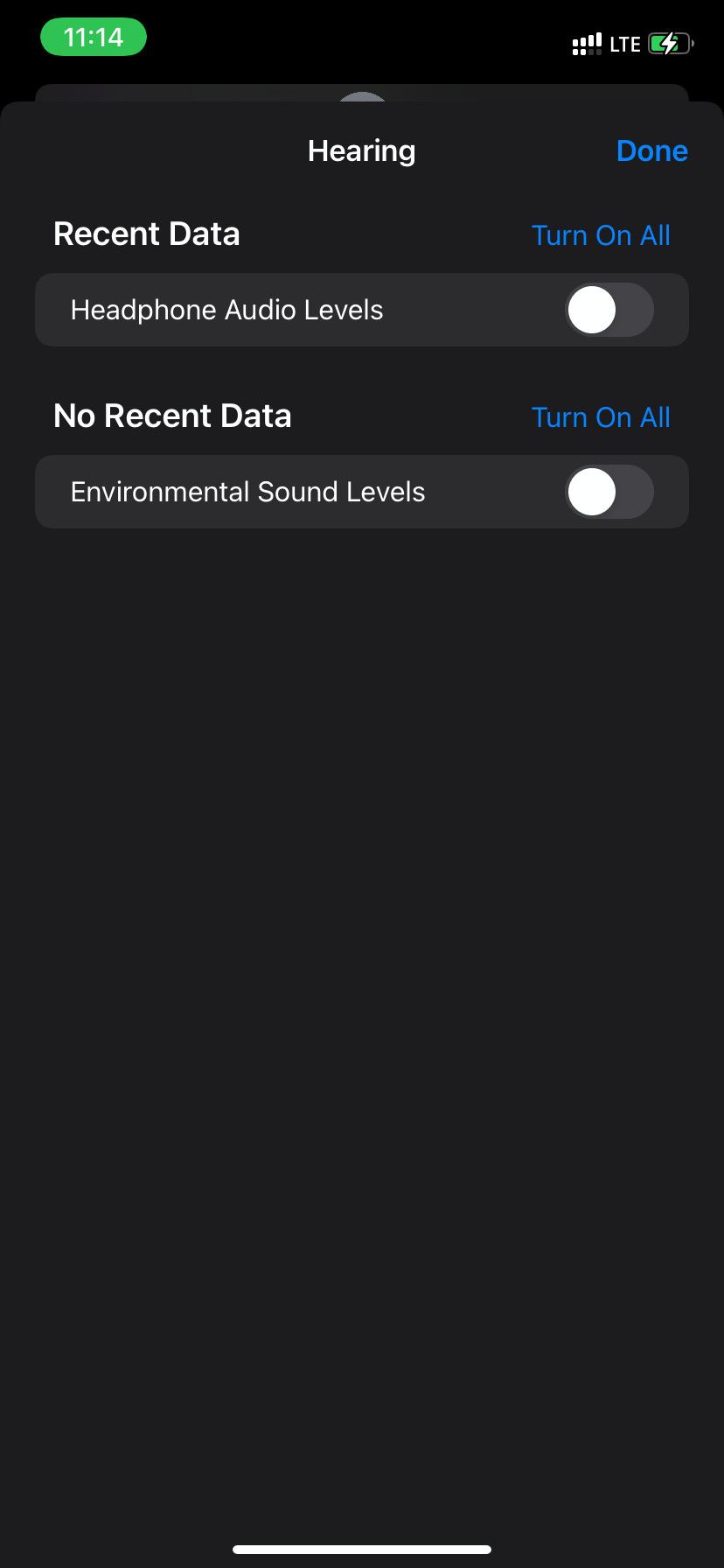A screenshot of an iPhone interface displays the 'Hearing' settings within the accessibility options. In the top-left corner, a green notification bubble shows the time as 11:14, while the top-right corner indicates a strong LTE signal with four bars and a battery icon that includes a charging symbol.

The main part of the screen is predominantly dark, utilizing a night or black theme with white text. At the top-center of the screen, 'Hearing' is prominently displayed with a 'Done' button to the right. Below, the interface is segmented into various sections. The 'Recent Data' header appears with a 'Turn On All' toggle to the right, both currently inactive. The 'Headphone Audio Levels' section follows, showing no recent data and an unchecked box beside 'Turn On All.' Further down, the 'Environmental Sound Levels' section also remains unchecked.

The bottom of the screen features the distinctive white bar of the iPhone home gesture, indicating that a swipe-up action will return the user to the home screen. The screenshot is characteristic of a straightforward, minimalist design with no people or additional imagery, solely focusing on the detailed display of the hearing settings.